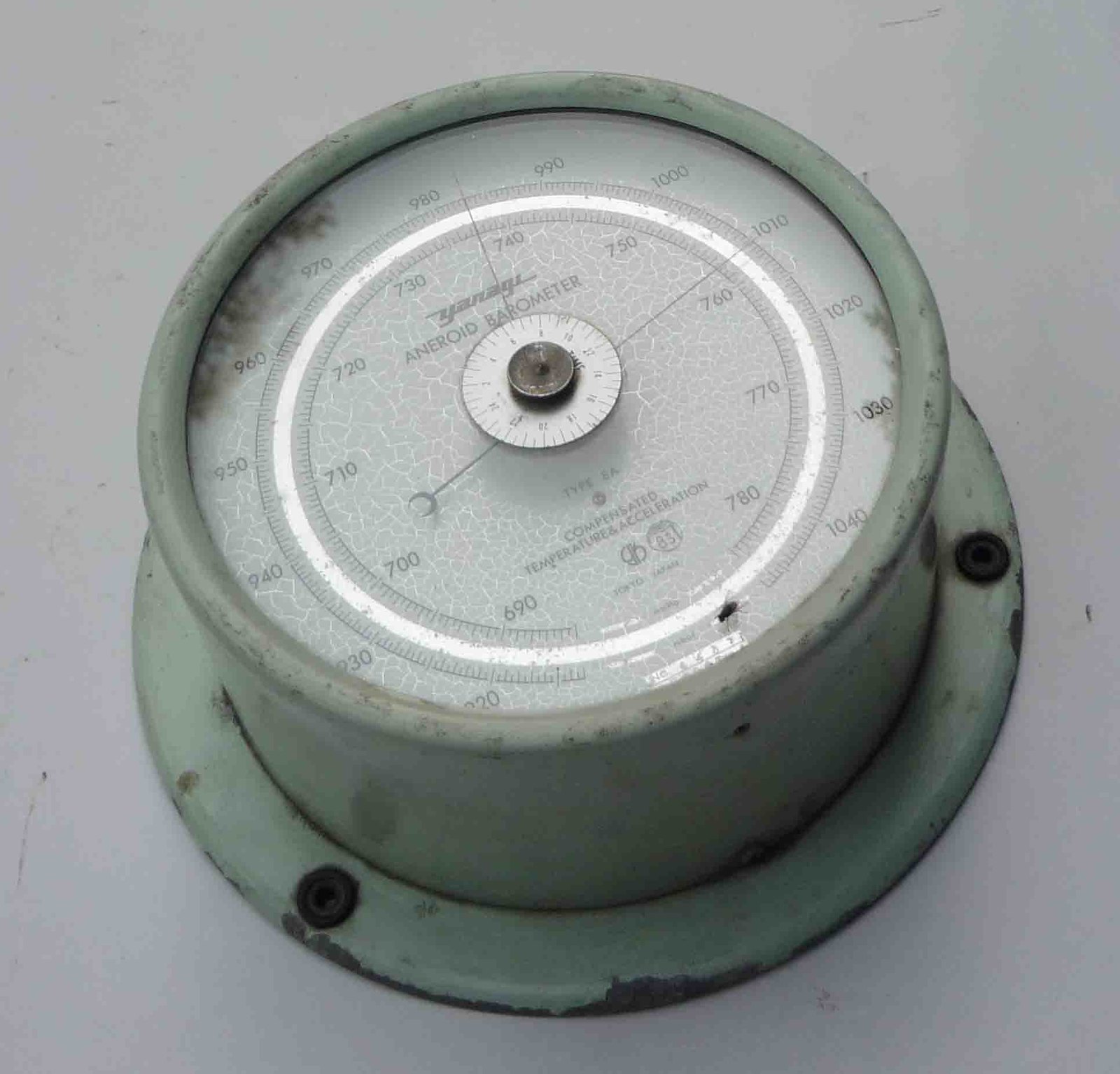The image features an antique aneroid barometer, characterized by its circular clock-like shape. The device has a complex dial system consisting of inner and outer circles marked with various numerical values. The inner circle displays pressure measurements ranging from 690 to 780, increasing by tens. The outer circle is graduated from 920 to 1040, also in increments of ten, encircling the entire face of the barometer.

In the center of the device, the phrase "Compensated Temperature Acceleration" is prominently inscribed, indicating a specific calibration feature. The top of the barometer bears the label "Aneroid Barometer," signifying its type. The instrument shows signs of considerable age, with its exterior exhibiting rust and an old, weathered appearance. Notably, there are signs of peeling at the bottom, further suggesting its vintage status. The barometer features a distinctive lime-green coloration, contributing to its aged and somewhat rustic charm.